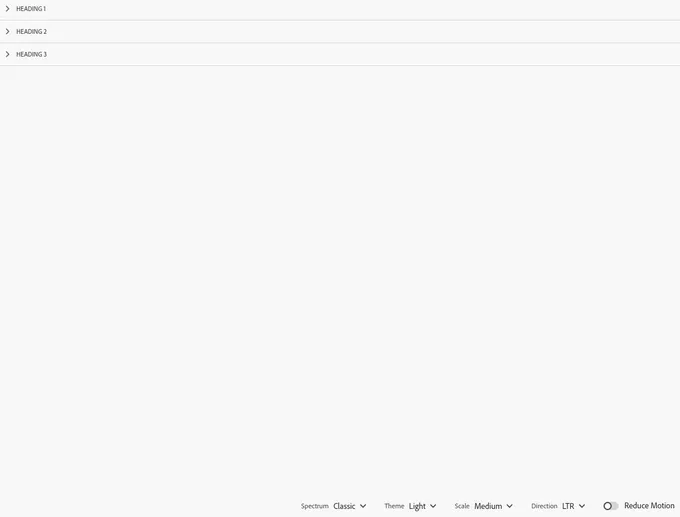Image Description:

The image displays a web page in landscape orientation, as seen on a laptop screen or monitor. The screenshot is somewhat blurry but shows a primarily blank, white background. Across the top are three thin, gray horizontal lines, collectively taking up about an eighth of the page.

- Along the first line, there is a label "Heading 1" with an open, right-pointing arrow (similar to a "V" turned on its side) to the left of the text.
- The second line similarly features "Heading 2" with a right-pointing arrow.
- The third line shows "Heading 3" with yet another right-pointing arrow.

These headings suggest that you can click on the arrows to expand or collapse sections or possibly edit the headings.

The rest of the page is completely blank until you reach the bottom. Aligned toward the right at the bottom and extending over halfway across the page to the left are different categories:

1. "Spectrum" with the label "Classic" and an expansion drop-down arrow next to it.
2. "Theme" which says "Light" with an arrow next to it, indicating the option to possibly switch to a dark theme.
3. "Scale" marked as "Medium" with an arrow, suggesting adjustable scaling options.
4. "LTR" (likely referring to text direction as Left-To-Right) with an arrow hinting at customizable text direction preferences.
5. "Reduce Motion" accompanied by an icon resembling a vibrating circle, implying a setting to reduce motion effects.

Overall, the web page appears to be an interface for customizing settings, likely related to photo or image editing based on the context provided.